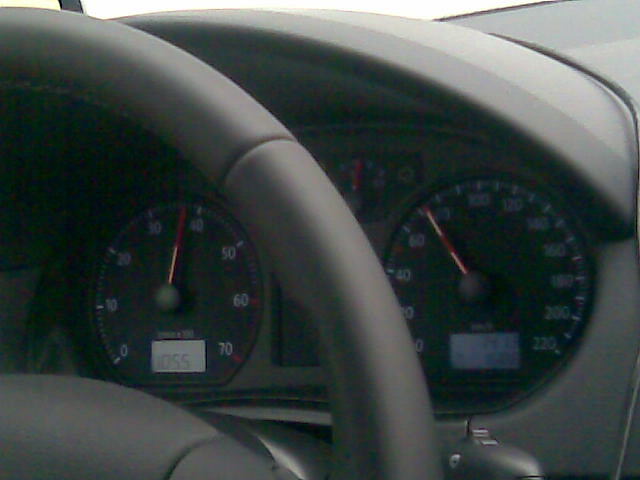This color photograph offers an intimate close-up of a car's interior, focusing predominantly on the steering wheel and dashboard. Viewed from a slightly right-side angle, the medium gray steering wheel commands attention as it arcs from the upper left corner of the frame, descending towards the bottom center. The dashboard accompanies the wheel, showcasing two prominent analog dials. 

On the left, the speedometer stands out, marked with regular increments up to 70 mph, each numeral sharply defined. A thin red needle accentuates the dial, pointing to the current speed. The right-side dial densely populates with numbers escalating to 300, though its exact purpose is less clear. This dial also features a central knob and a red hand indicating its metrics.

Centrally positioned above the steering wheel's edge, another dial emerges but remains blurred and unreadable, adding a hint of mystery to the otherwise clear and detailed instrumentation. The photograph's tight composition and focused detailing encapsulate the intricate functionality and design elements of the vehicle's dashboard.